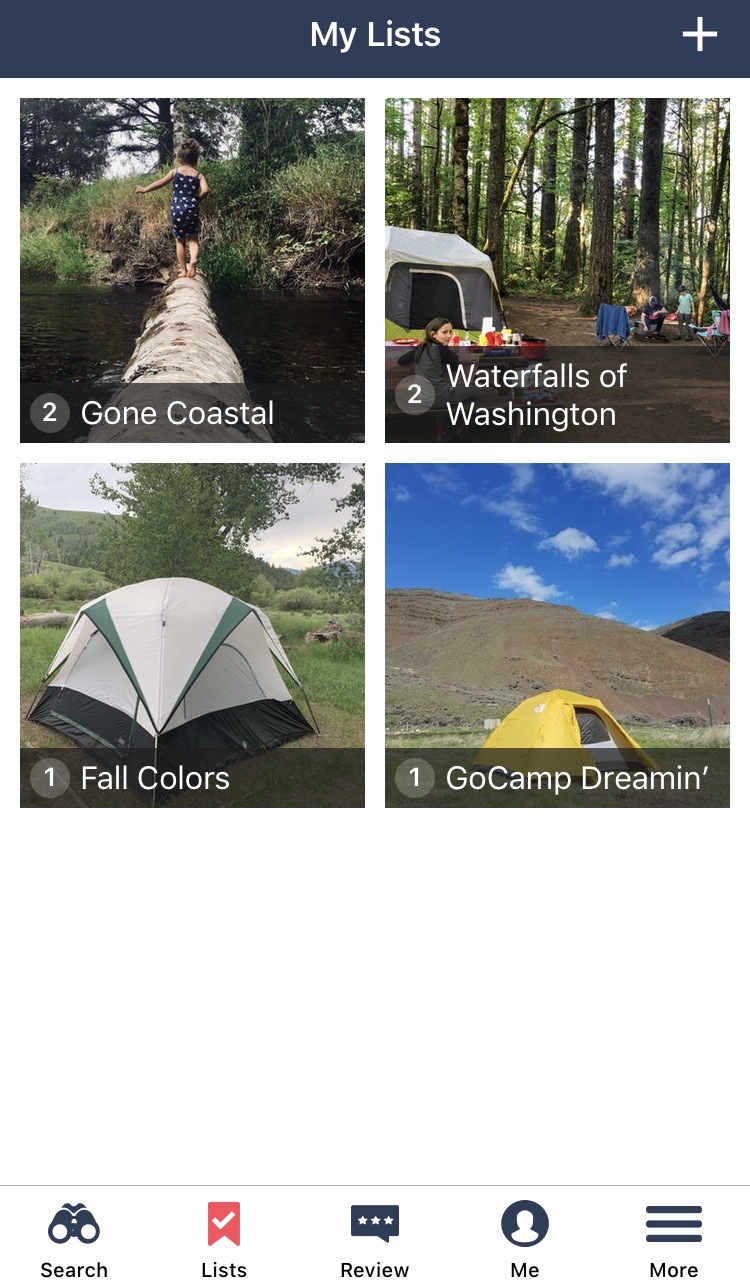The image features a navy blue banner at the top, centered with the text "My List" in white. In the upper right-hand corner of the banner, there is a white plus sign. Below the banner, the image is divided into four squares, each containing a distinct photograph and a circular number followed by a short description.

In the top left square, there is a picture of a forested area with a log spanning a river or stream. A little girl is walking across the log. Below this image, there is a circular number "2" followed by the text "Gone Coastal."

The top right square showcases a campsite. This scene includes a family near a tent, a picnic table laden with items, and people gathered around a fire pit with camp chairs. Tall forest trees provide the background. The circular number "2" is located below this photo, along with the text "Waterfalls of Washington."

In the bottom left square, there is an image of a tent pitched in a meadowed area surrounded by trees. This photo is labeled with a circular number "1" and the text "Fall Colors."

The bottom right square displays a tent in a deserty, hilly landscape under a blue sky with clouds. The caption below features a circular number "1" followed by the text "Go Camp Dreaming."

At the bottom of the entire image is a horizontal line under which there are five different symbols, each followed by a word. From left to right, the symbols are:
1. Binoculars with the word "Search"
2. A list with the word "Review"
3. A page with the word "Review"
4. A person with the word "Me"
5. Three dots with the word "More"

Each symbol is aligned above its respective word.